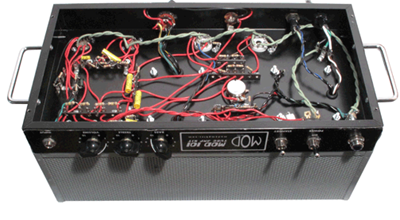This color photograph features a detailed close-up view of an audio speaker or amplifier, placed upside down on a white background, with the top panel removed to expose its intricate internal wiring. The outer casing of the speaker has a black top and side panels, and the front part features a gray mesh grille. Visible on the front are several black control knobs, six in total, with three on each side of an upside-down brand label that appears to read "MOD." The knobs have white dial markings and are set in a row. On either side, there are silver handles, providing grip for carrying. The internal components revealed by the removed top panel include an array of red, blue, white, and turquoise wires, zigzagging across a black surface. Additionally, there are yellow fuses and a circuit board to which the wires are connected. No external electrical cables, people, animals, or other structures are visible in this photograph.